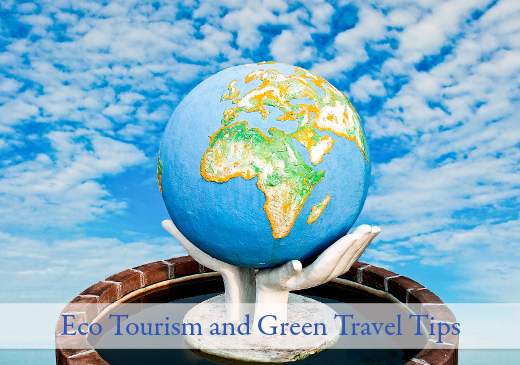The image depicts a serene blue sky filled with white, wispy cirrus clouds. At the center of the picture is a detailed globe, showcasing the blue oceans and the continents of Africa, Europe, and parts of Asia, highlighted in green and yellow. The globe is held aloft by two white hands, sculpted to appear as though they are gently cradling it. These hands are positioned atop a circular stand bordered with red bricks that are meticulously lined with white cement. At the bottom of the image, a white band with blue text prominently displays the words "ecotourism and green travel tips." This visually striking arrangement suggests an educational or promotional theme likely related to travel or environmental sustainability.